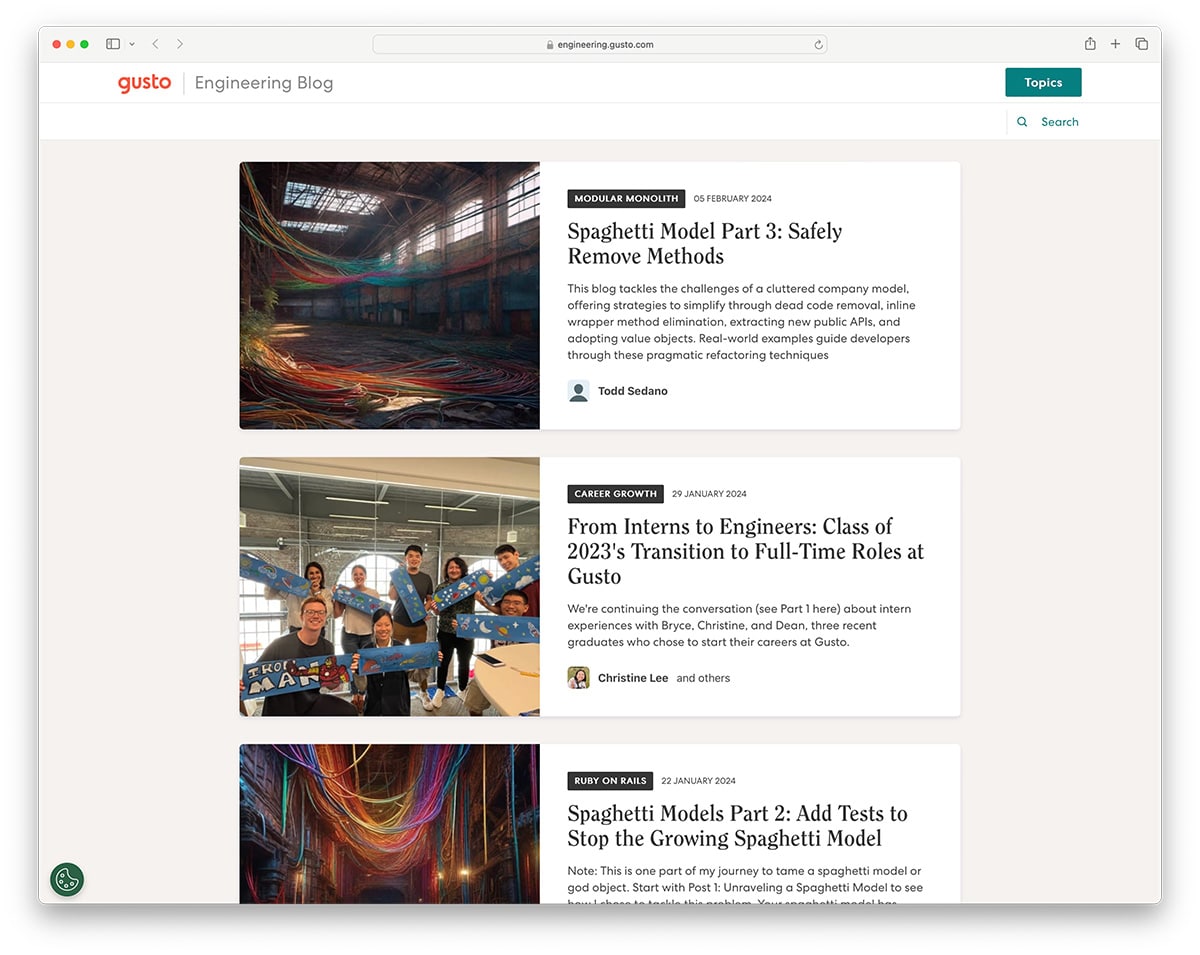This cropped screenshot captures a segment of a desktop browser displaying the Gusto Engineering Blog. In the top-left corner, the word "Gusto" is prominently featured in lowercase red letters. Immediately to its right, "Engineering Blog" is displayed in large grey font. Adjacent to this, a green box marked "Topics" in large white letters is visible. Below this box, there's a search icon accompanied by the word "search" in green text.

The background beneath the header transitions to grey, showcasing a vertical list of articles. The foremost article includes a large square thumbnail image on the left. To the right of this image, the article title "Spaghetti Model Part 3: Sexily Removed Methods" is prominently displayed in bold black font. A brief description follows underneath the title. At the bottom left of this article preview, the author's profile photo and name are visible. Two additional articles are partially visible, with the third article requiring further scrolling to view in its entirety.